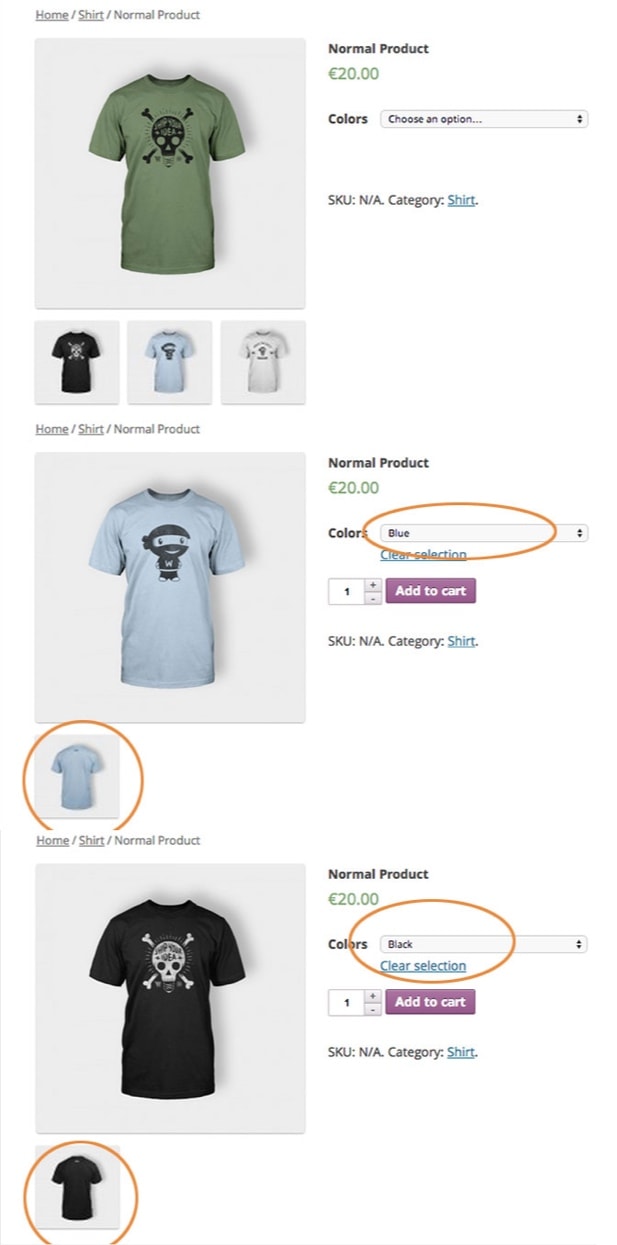The image is a screenshot of an e-commerce webpage featuring a selection of t-shirts. At the top of the page, the navigation menu is visible with the following options: "Home," "Shirt," and "Normal Product." The "Normal Product" category is currently highlighted, while "Home" and "Shirt" have underlines beneath them, indicating they can be selected.

Below the navigation bar, there is a section displaying a specific t-shirt product. The t-shirt in question is shown inside a square and features a graphic of a skeleton with a poison symbol. To the right of this image, the product is labeled "Normal Product" with a price tag of 20 euros. Below the price, there is an input box labeled "Choose an option" for selecting different colors. The product information further includes an SKU listed as "N/A" and the category "Shirt," which is presented as a clickable blue button.

Under this section, there are visual options for three different t-shirt colors. Below these options, another t-shirt is displayed: a blue t-shirt featuring a ninja and animation design. Following this is an image of another t-shirt in black, also adorned with a poison symbol. Alongside each t-shirt image, there are details including the product name, price in euros, available colors, and options for selecting the quantity to add to the cart.